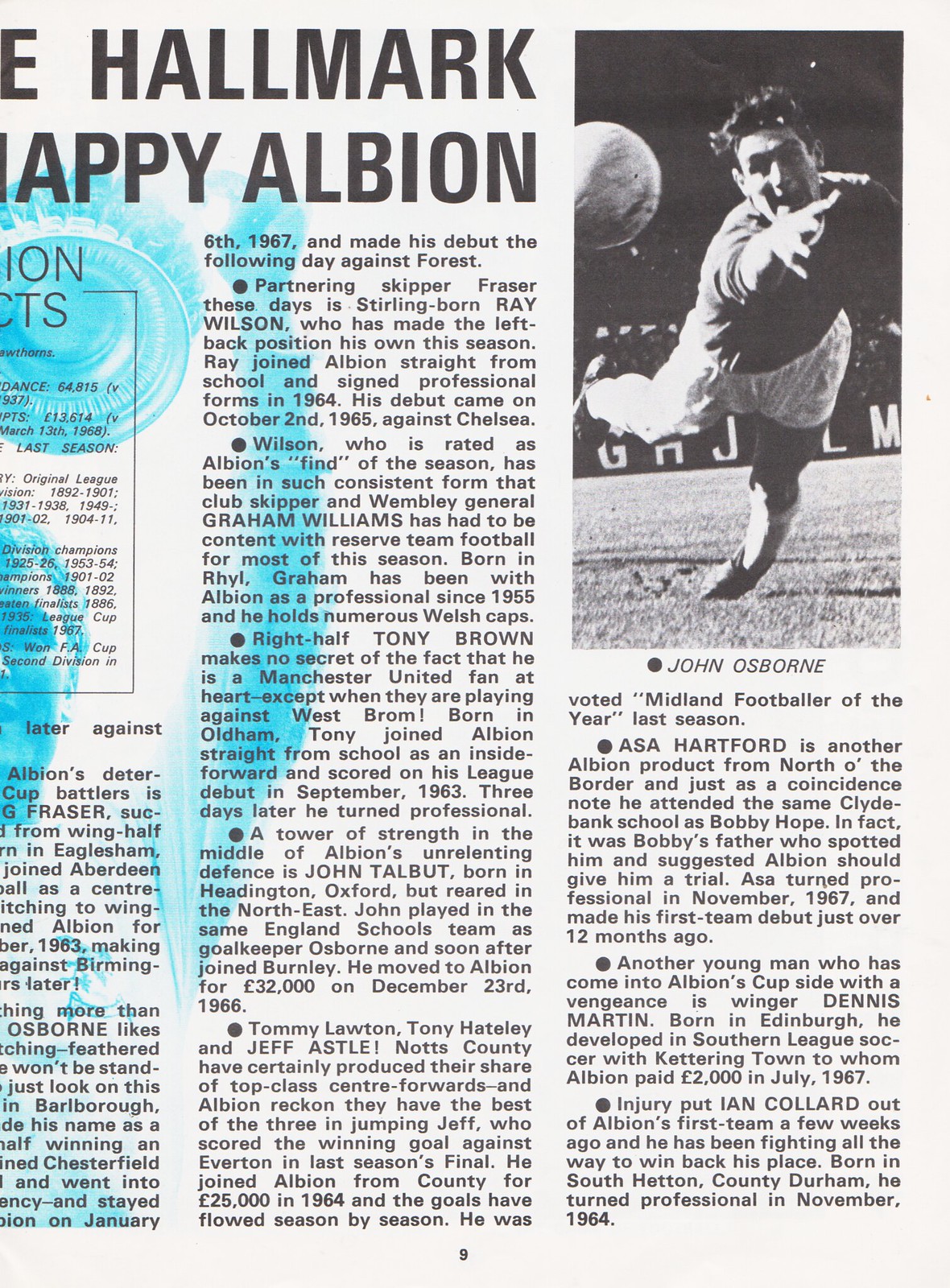This is a historical newspaper article from 1967 featuring John Osborne, a noted soccer player. The article, adorned with a black-and-white photograph of Osborne leaping to catch a ball, suggests he was a goalie. The photo is an archival image adding a nostalgic touch. The article provides extensive coverage of various players from the team over the years, detailing their careers and significant games. Despite some parts of the article being cut off, we learn that Osborne made his debut with Hallmark Albion, with other notable players like Ray Wilson also mentioned. The article is stained with blue ink, possibly from a stamp or spill, lending it an authentic, aged appearance. Overall, it offers a rich historical perspective on the careers and achievements of several soccer players.